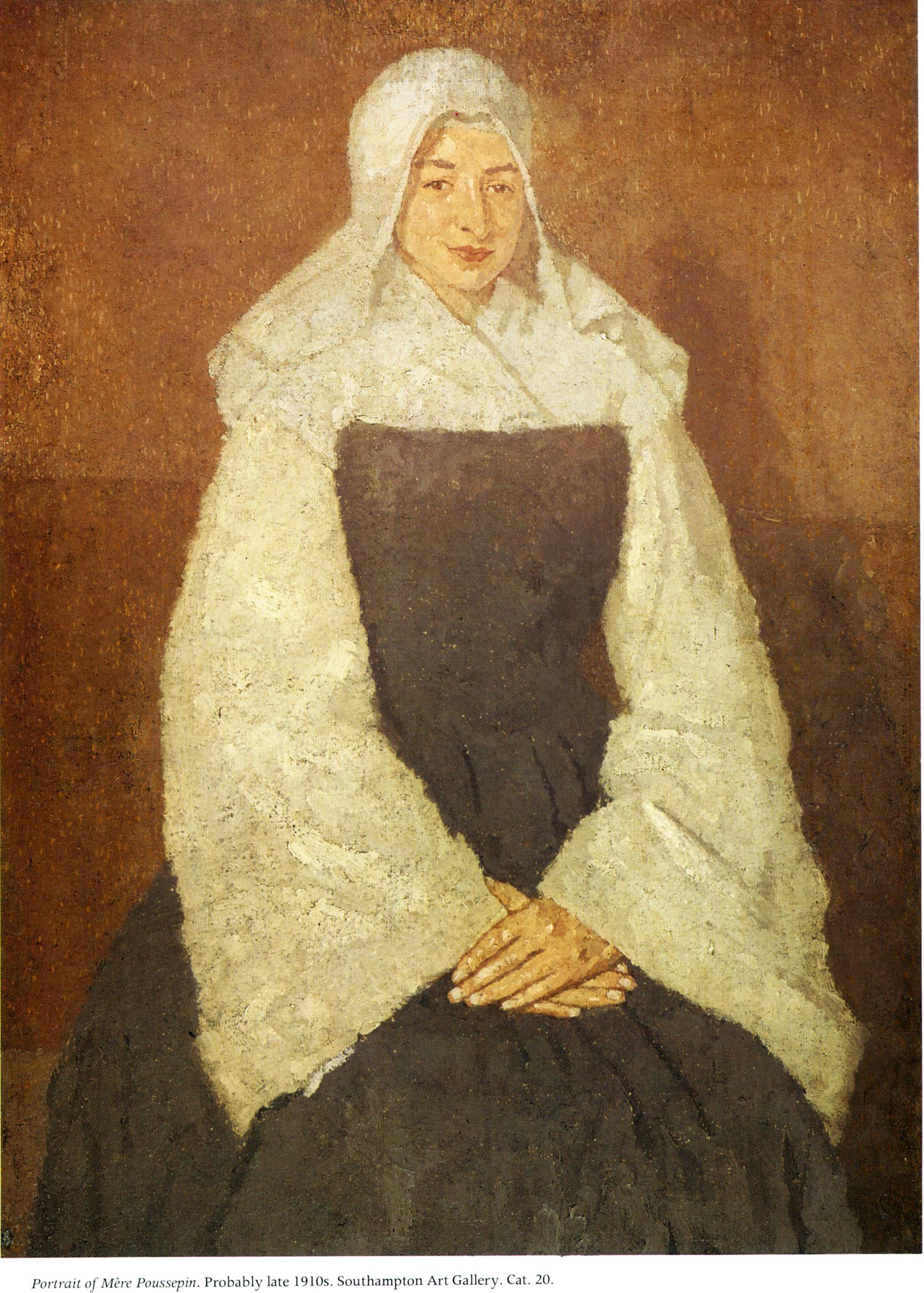The image depicts a very old painting featuring a woman seated prominently in the center against a background that transitions from dark umber to a lighter tan shade. The woman, slightly smiling, wears a long black dress with a white shawl collar and wide white sleeves that extend to her wrists, where her hands are shown clasped together in her lap. Her head is covered with a white headscarf. She has dark eyes, dark eyebrows, and pinkish lips with a slight yellowish skin tone. The bottom of the image is captioned "Portrait of Mère Poussépin, possibly late 1910s, Southampton Art Gallery, CAT 20."